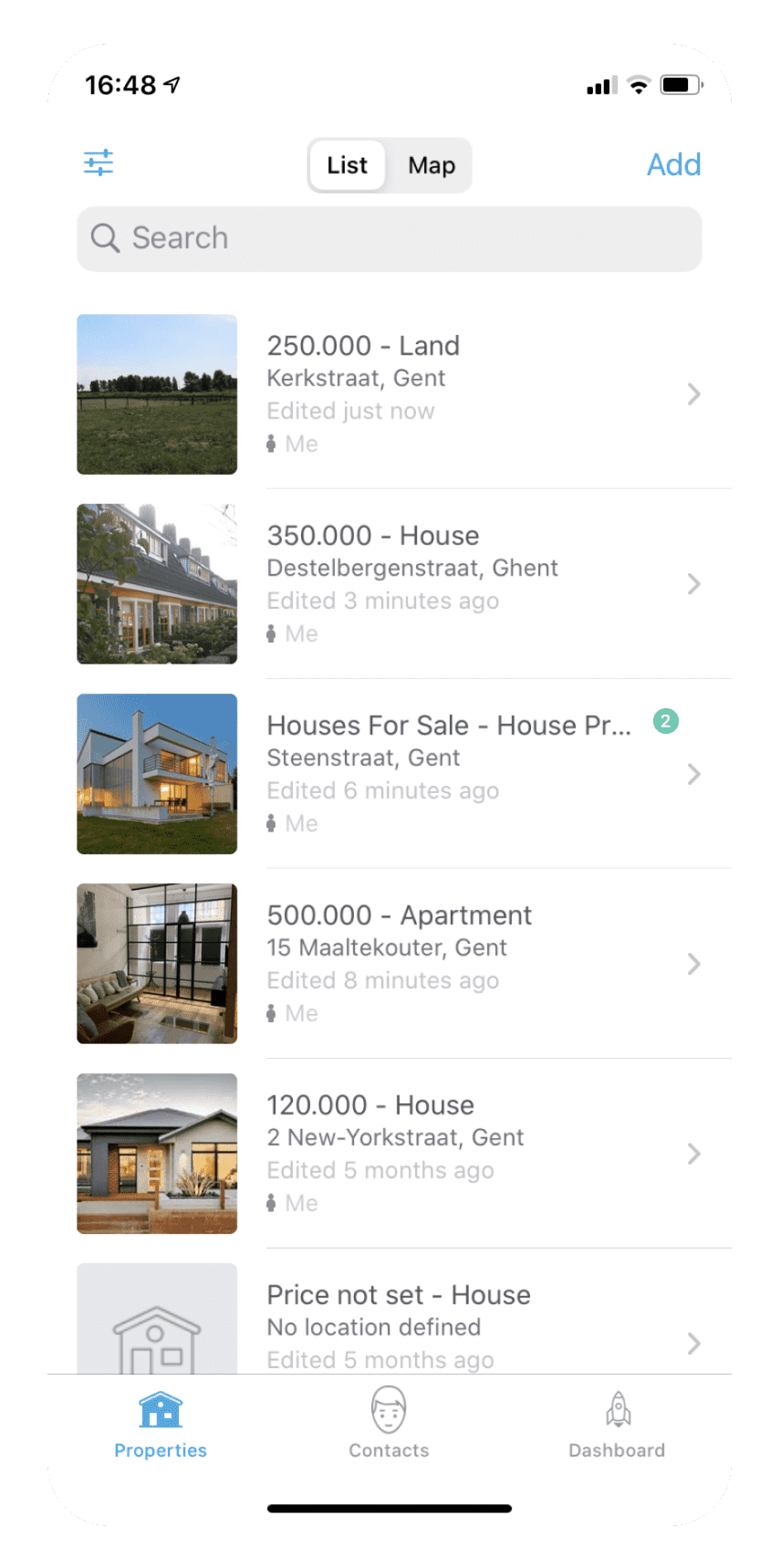The image depicts a list of homes available from the year 1648, displayed on a white rectangular section against a gray background. The interface features a search bar at the top, accompanied by a blue "Add" button.

The list includes different properties with the following details:
1. A plot of land priced at $250,000.
2. A house priced at $350,000, represented by a standard house image. Each item has a greater-than symbol to its right indicating more information can be accessed.
3. A 'houses for sale' section with a truncated description ("house pr…") and a small icon displaying the number '2' inside a green circle.
4. An interior view of a house followed by an apartment listed at $500,000.
5. A house listed at $120,000, described with the term "to move your" and the obscure location "Y-o-r-k-s-t-r-a-a-t, Gent."
6. A sketch of a house with "Price not set - house," suggesting it is not a real property but rather a placeholder image.

Each property is accompanied by relevant visuals such as photographs or sketches, enhancing the user experience.